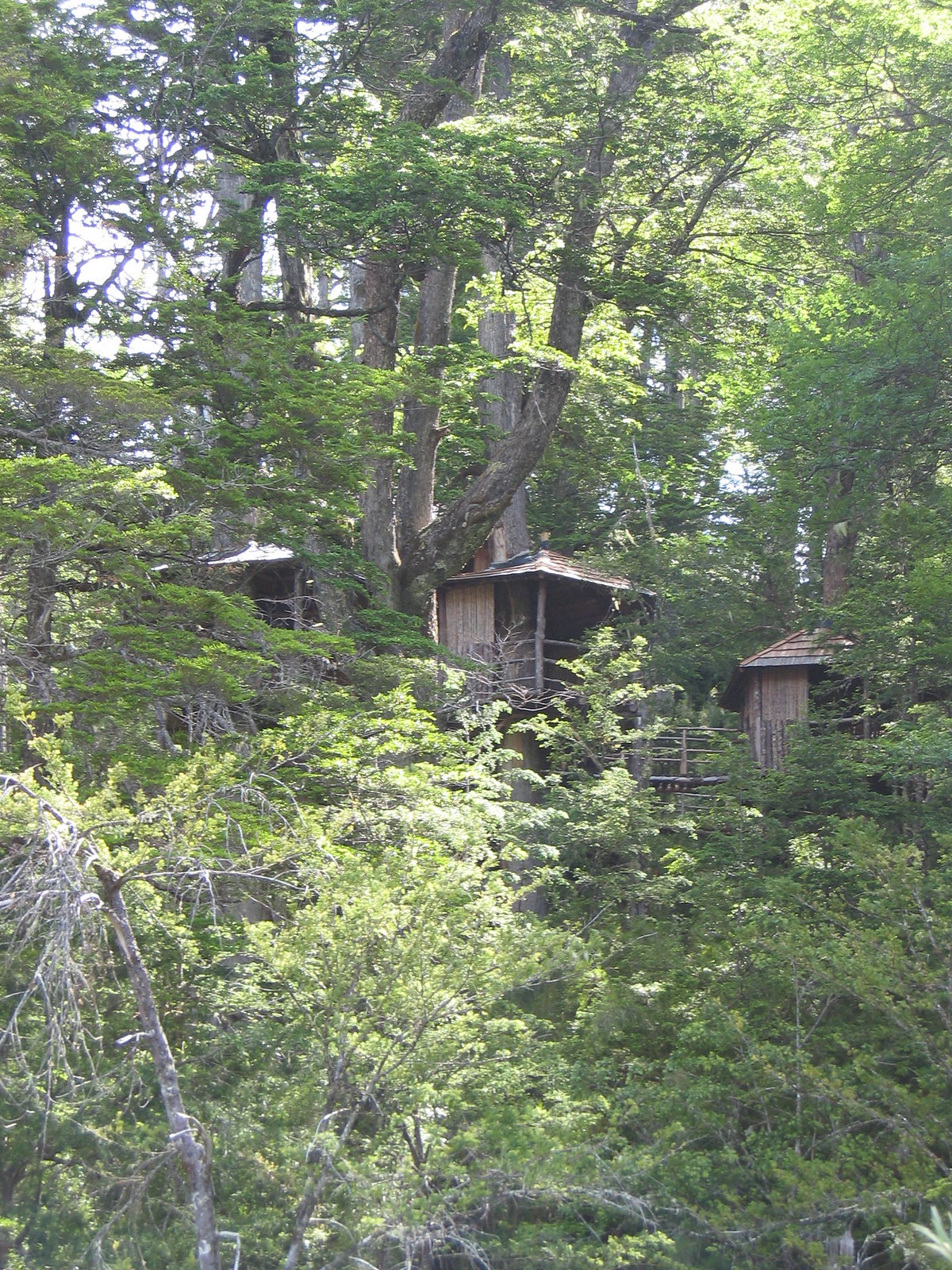The photograph captures a serene and adventurous daytime scene deep within a lush forest. Dominating the image are brown tree trunks and branches, blanketed in vibrant green leaves that allow rays of bright sunlight to filter through. Nestled high among the foliage are three simply constructed, square-shaped wooden tree houses, each distinguished by their triangular roofs. Elevated and interlinked by rustic wooden walkways, these tree houses exude a sense of a peaceful yet thrilling retreat, perhaps an eco-hotel or glamping location. The viewpoint of the photo, taken from one of these elevated dwellings, offers a unique vantage over this enchanting arboreal hideaway.